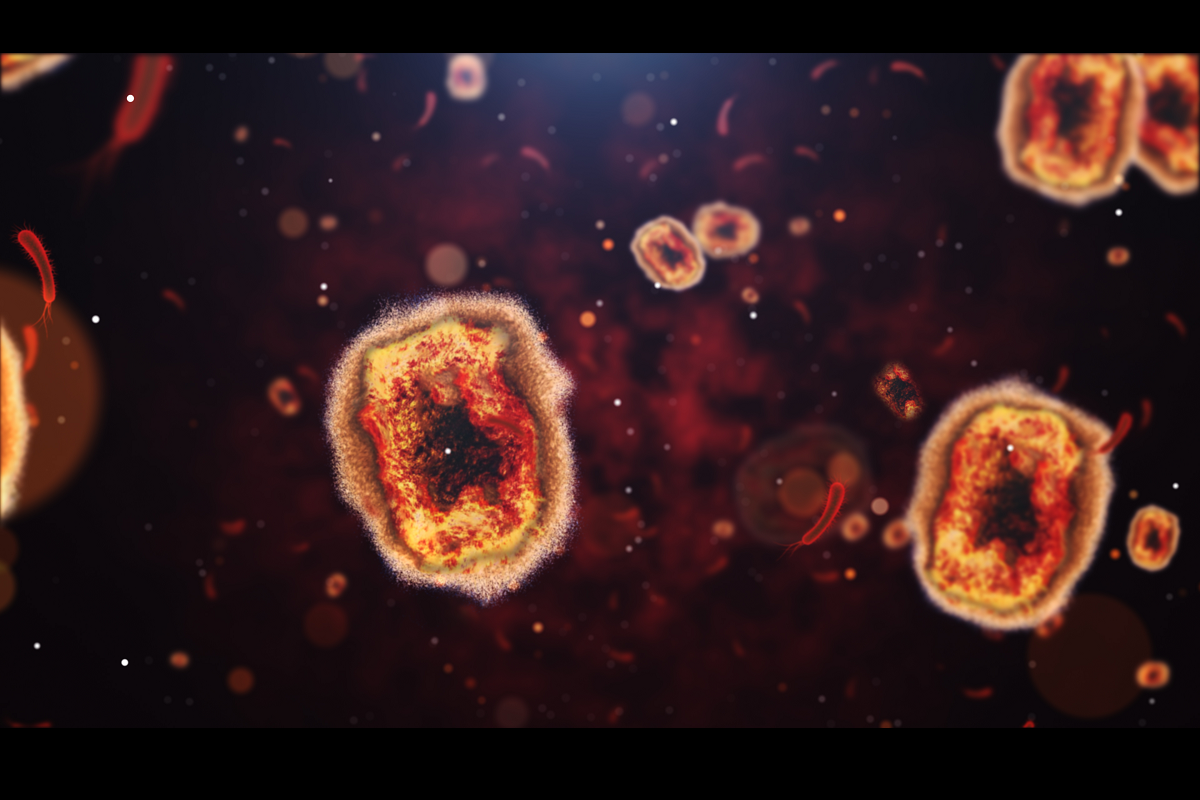This photographic image, possibly taken through a microscope, depicts six prominent cells against a maroon and black background with orange splotches. Each cell features a distinct structure: a brown cell wall with a dark brown border, enclosing an orange and yellow body with a central black nucleus. The cells are arranged in a pattern: two larger cells dominate the top right-hand corner, while the largest cell is situated at the center. To the left of the image are two smaller cells, each about a third the size of the central one, and the bottom right-hand corner hosts a cell comparable in size to the central cell. The background is maroon with black undertones, devoid of any text. The arrangement and clarity of the cells suggest a scientific or classroom setting, possibly resembling a zoomed-in image of blood cells, with some cells appearing more faded as they recede into the background.